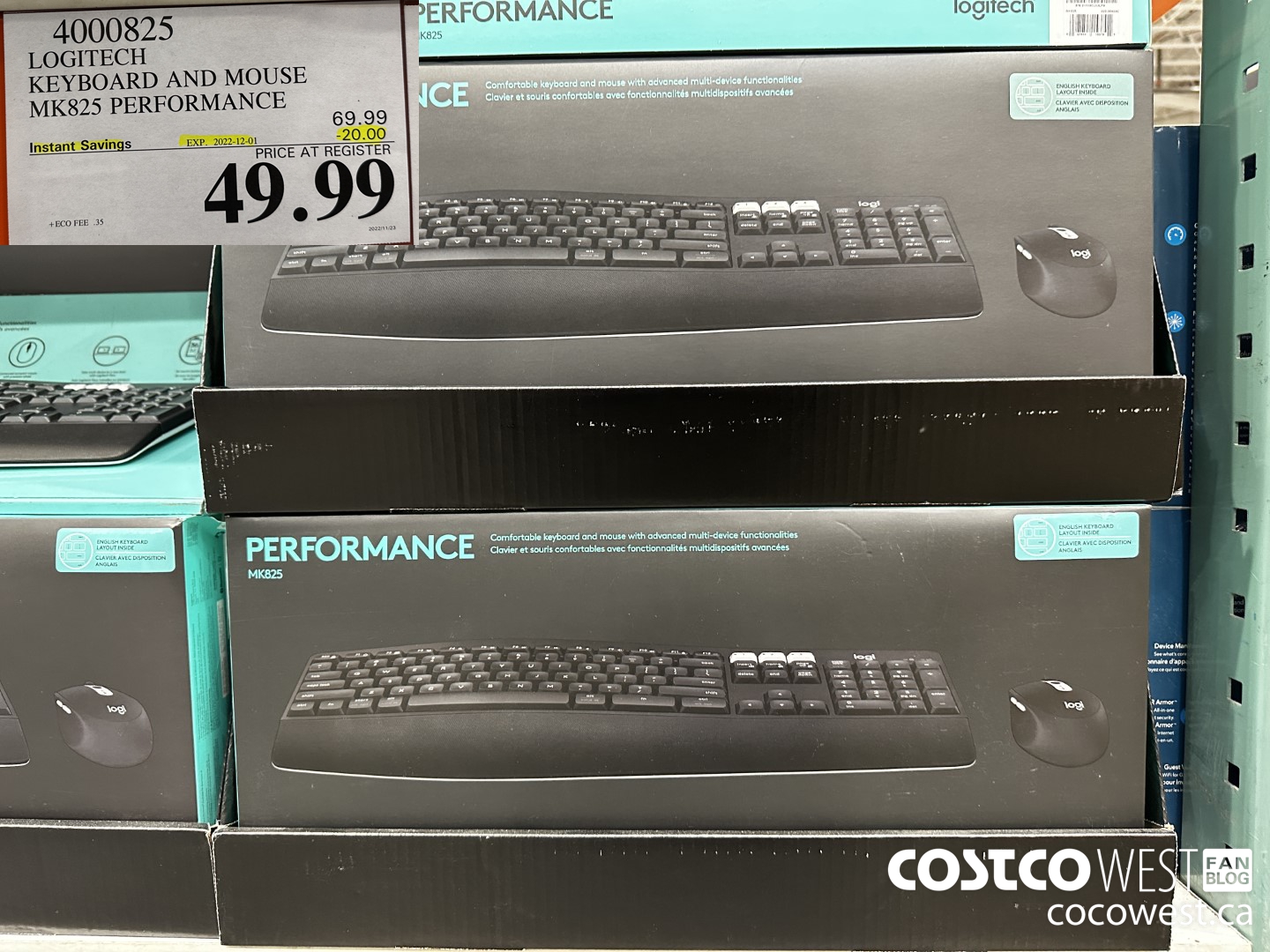**Caption:**

In this detailed image, we see a Logitech mouse and keyboard combo, specifically the MK825 performance model, packaged in a box predominantly colored in black and teal green. The box features an image of the sleek black keyboard and mouse prominently on its front side. On the upper left corner of the image, there is a black and white pricing label. It indicates an instant savings offer of $20 off the original price of $69.99, reducing the price to $49.99.

The setting appears to be a store, most likely Costco, as suggested by the label on the bottom right corner that reads "Costco West Fan Blog, Coco Walnut, California". The image shows multiple stacked boxes of the same Logitech combo on the left and center sections, while the right side features part of a green-colored shelf. The overall composition effectively showcases the product alongside its current promotional offer.